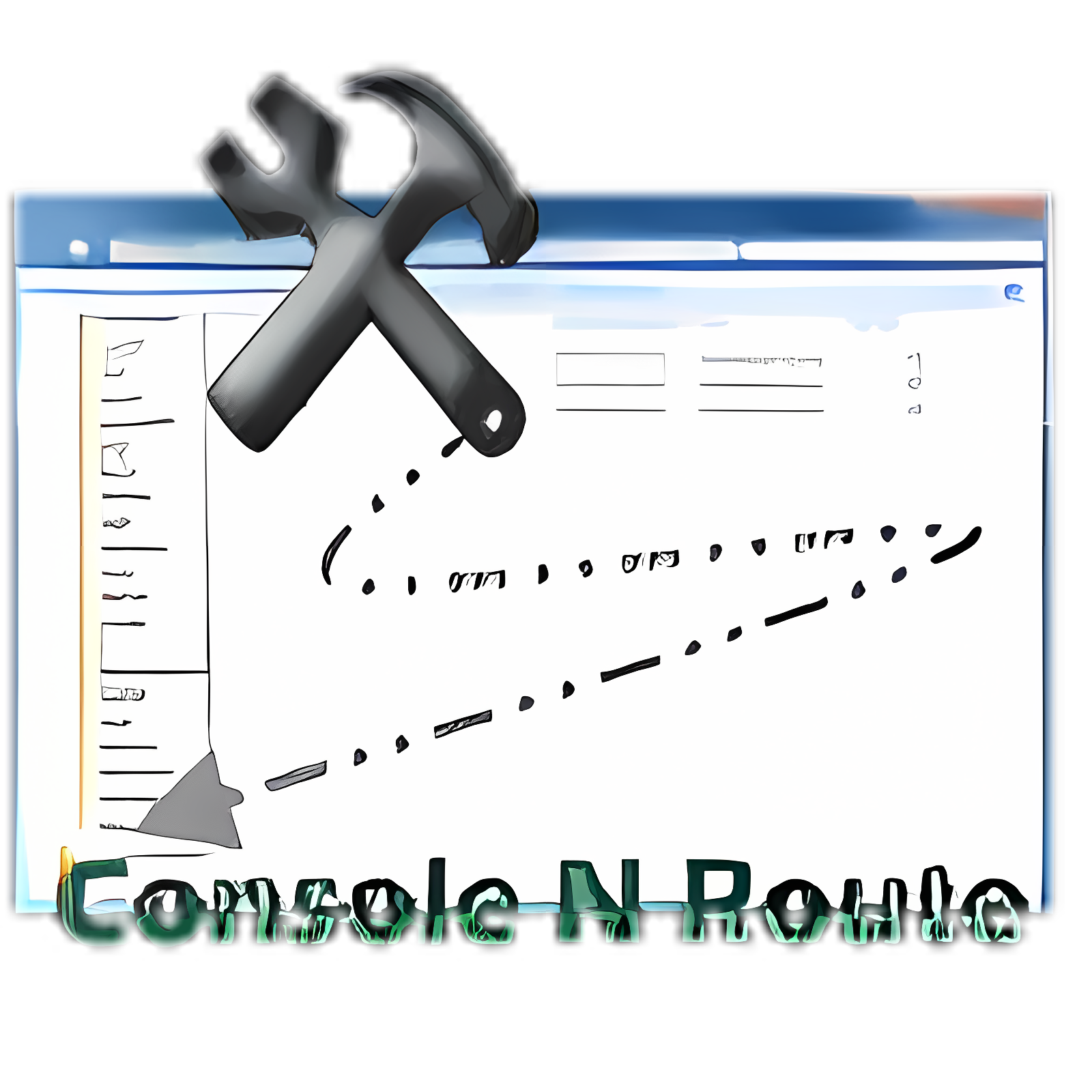The image is a crude illustration of a web page or report with a blue banner at the top that fades into white. In the center, there are two tools, a black hammer and wrench, forming an X shape. The background includes various indiscernible lines and figures, creating a scribbled look. On the left side, there is a vertical column of scribbles. In the upper center and upper right, there are several boxes filled with more scribbles. A dotted and dashed line originates from one of the tool handles, curving down and around the page, culminating in a gray arrowhead in the bottom left corner. Beneath this entire scene, there's text in a fuzzy green font that appears to read "CONSOLENRULE."